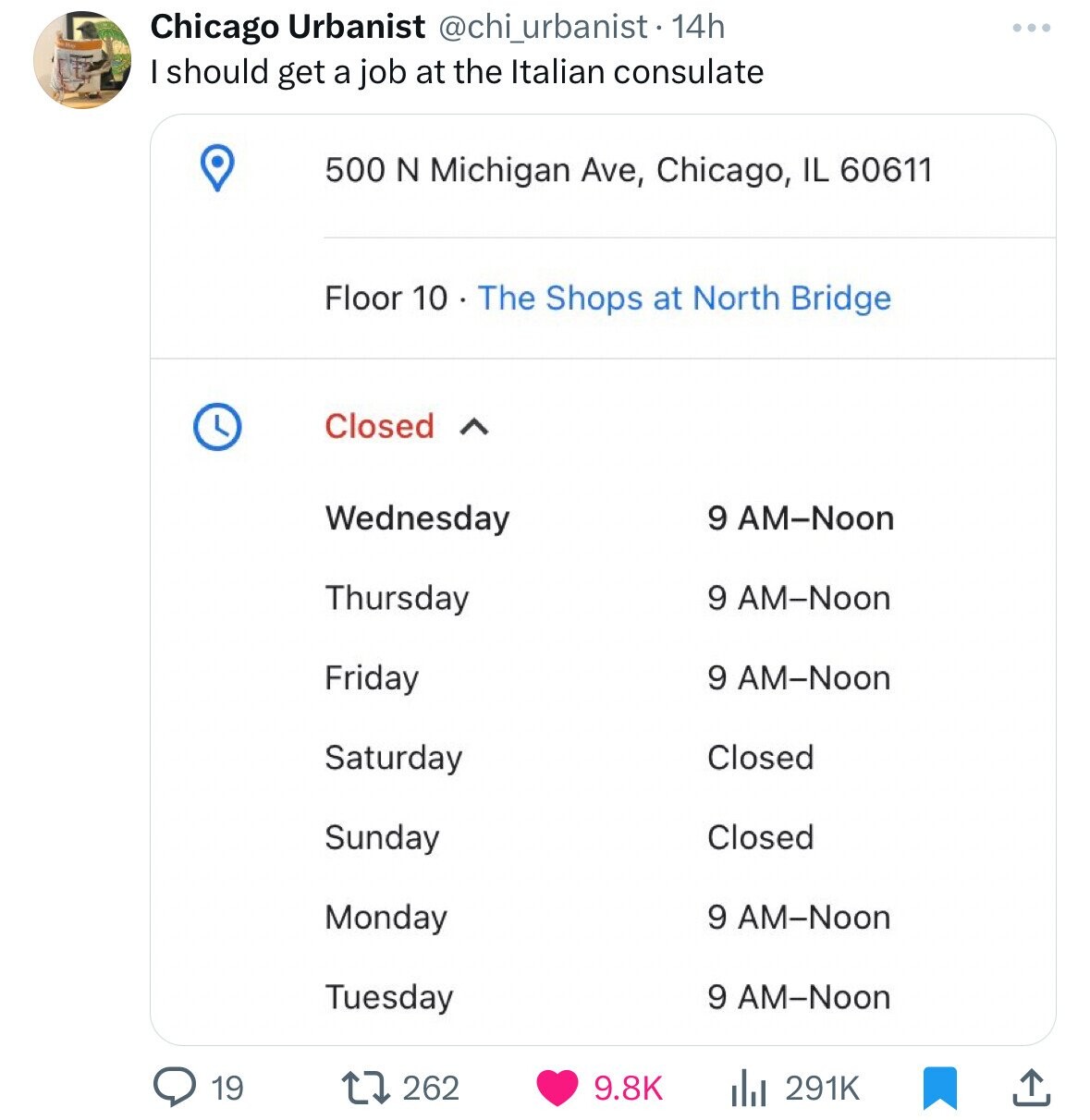Here is a detailed caption for the screenshot:

---

**Screenshot of Chicago Urbanist Social Media Post**

**Title:** Chicago Urbanist  
**Handle:** @chai_urbanist  
**Post Time:** 14 hours ago

**Content:**  
“I should get a job at the Italian Consulate.”

**Details:**  
**Address:**  
500 North Michigan Avenue,  
Chicago, Illinois IL 60611

**Location:**  
10th Floor, The Shops at North Bridge  

**Business Hours:**  
- Closed  
- Wednesday: 9 AM - Noon  
- Thursday: 9 AM - Noon  
- Friday: 9 AM - Noon  
- Saturday: Closed  
- Sunday: Closed  
- Monday: 9 AM - Noon  
- Tuesday: 9 AM - Noon

**Post Statistics:**  
- Comments: 19  
- Shares: 262  
- Likes: 9.8k  
- Views: 291k  
- Saved: 
- Direct Messages: